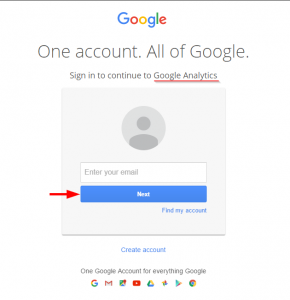A screenshot of a Google sign-in page. The background is predominantly white. At the top, the colorful Google logo is displayed, followed by the text, "One account. All of Google." Below it, the prompt reads, "Sign in to continue to Google Analytics," with a distinctive red underline emphasizing "Google Analytics."

Next, there's a gray box that includes a gray circle featuring a stylized user icon, symbolizing a profile. The instruction "Enter your email" is written next to it. A red arrow points to a blue button labeled "Next." Beneath this button, there's a smaller blue text link stating, "Find my account." Another blue link follows, reading, "Create account." At the bottom, the text, "One Google account for everything Google," reiterates the unified nature of Google's services.